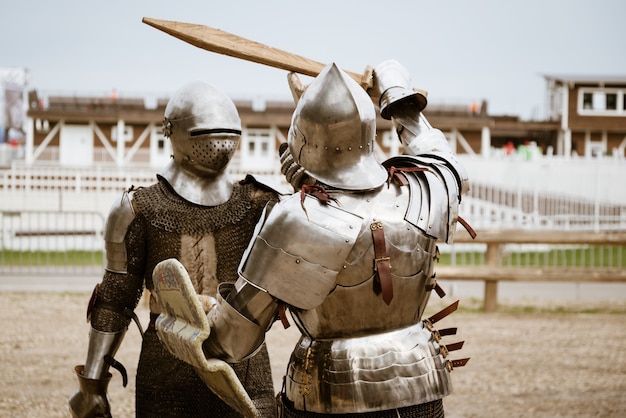In this vintage-looking photograph, we see two individuals dressed as knights, engaging in a mock duel with wooden weapons. The knight on the left is clad in full plated armor with a pointed helmet and is holding a wooden sword high in the air. The other knight, facing him, wears chain mail armor and is equipped with a wooden shield. They stand on a dirt ground enclosed by a wooden fence, beyond which lie barns with brown roofs and white wood porches. The scene appears to be set at a ranch or field, suggesting a reenactment event where modern-day enthusiasts mimic historical knightly combat. The knights, though not truly from the Middle Ages, look intently at each other, poised in their silverish armor and ready for their next move.